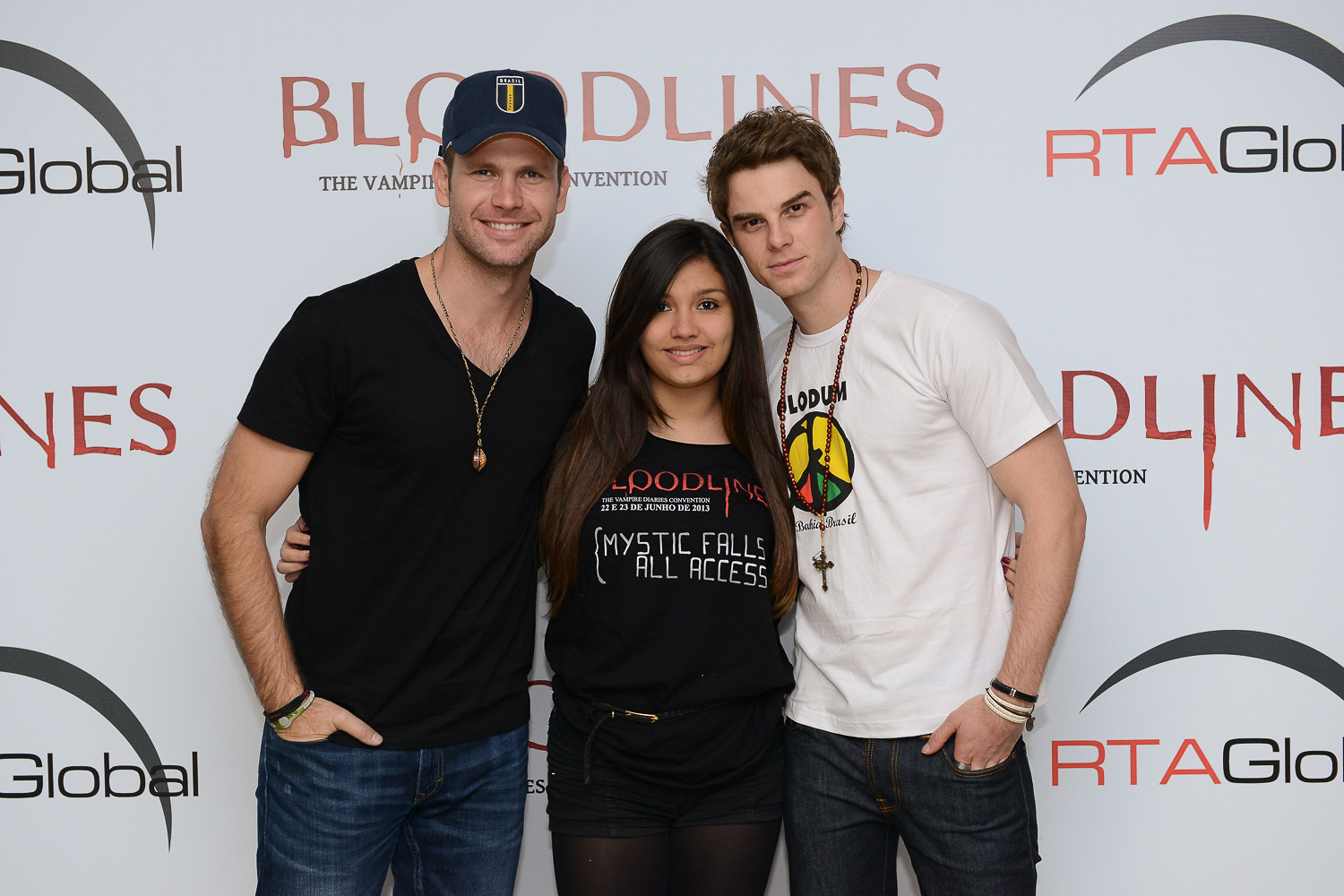The image depicts three people standing in front of a backdrop that partially reads "Bloodlines," "The Vampire Intervention," and "RTA," though the rest of the text is obstructed by heads and a logo. The setting is bright, possibly suggesting the photo was taken during the daytime, and the backdrop resembles those used at red carpet events or promotional interviews. On the left stands the tallest of the three, a Caucasian man with dark eyes and stubble, wearing a black V-neck t-shirt, blue jeans, and a black baseball cap. His right hand is in his pocket, and his left arm is around a woman in the middle. This woman, also Caucasian with long, shoulder-length hair and light-colored eyes, wears a black "Bloodline Mystic Falls All-Access" t-shirt and black shorts. To her right stands another Caucasian man with short dark hair, a white graphic t-shirt potentially displaying a peace sign or "Nolodun," dark jeans, and a cross necklace. All three appear to be posing for the camera, possibly as part of a promotional event for a TV series.